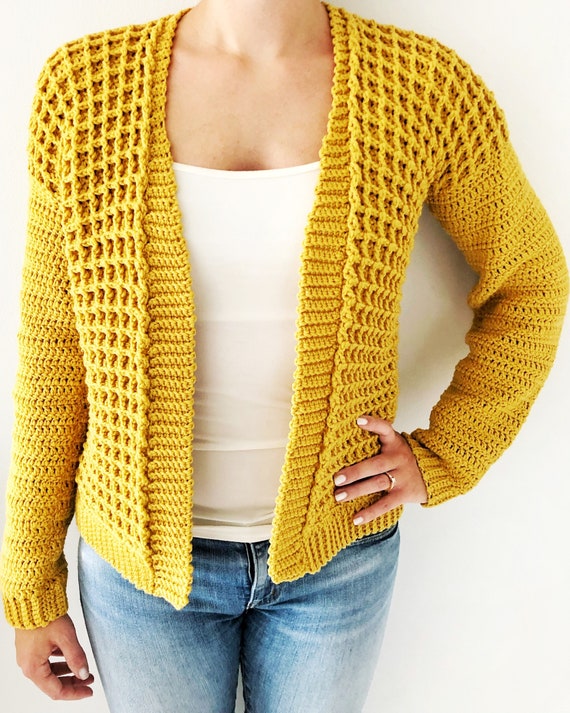In the image, a woman is showcased from the neck down to just above the knees, presenting a cozy, handmade mustard-yellow sweater with intricate square and block knitted patterns. The sweater features distinct ribbed cuffs and a hem, and it lacks buttons, allowing a glimpse of the tight-fitting, well-pressed white crop top she wears underneath. Her left hand, adorned with white nail polish and a wedding ring, rests confidently on her hip. Complementing her outfit are a pair of faded, blue jeans with an open button near the crotch. The scene is set against a subtle off-white wall, highlighting the craftsmanship and design of her sweater.